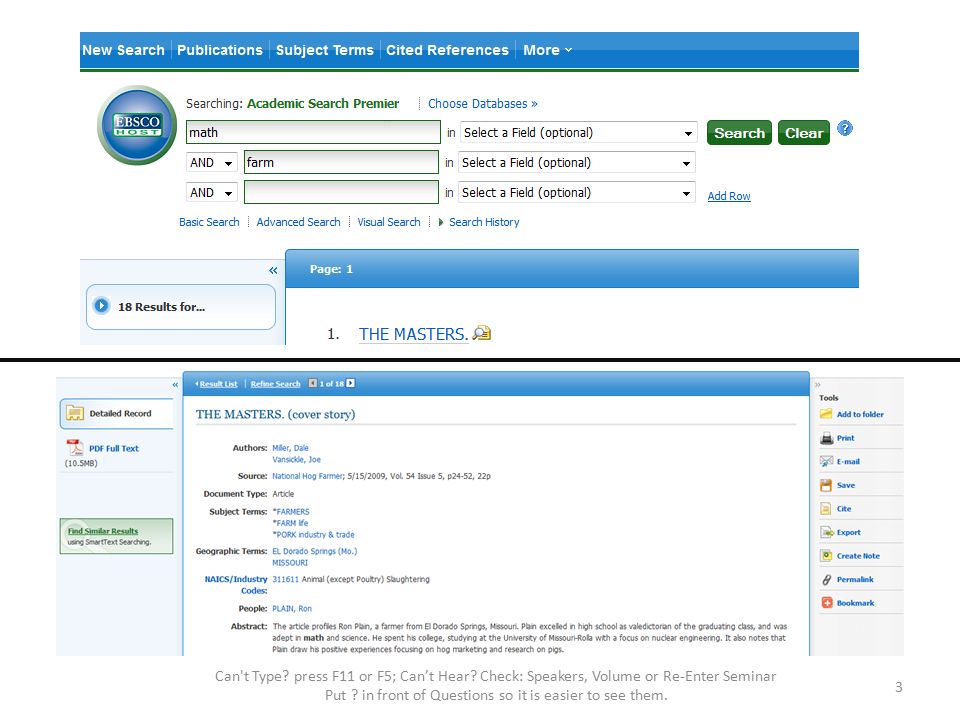The image features a predominantly white background interspersed with horizontal blue rectangular boxes. The topmost blue box has sharp edges and contains white text on the left side that reads "New Search." To the right of this, the box sequentially displays the words "Publications," "Subject Terms," "Cited References," and "More."

In the center of the image, there are two horizontally aligned blue rectangles with rounded edges. Within these rectangles, various input fields are displayed. The first text box on the left contains the word "Math," followed by another text box below it with the word "Pharm," and a blank text box beneath that. Adjacent to these are white boxes, each containing black text that reads "Select a Field."

Below these central elements is another blue rectangle on the left, featuring white text that states "Page" and the number "1." Further down, black text indicates "1." and blue text in all caps reads "THE MASTERS."

Another detailed rectangular blue box beneath this section is filled with informative text. The upper left of this box includes blue text in all caps, "THE MASTERS," followed by black text headers such as "Authors," "Source," "Document Type," "Subject Terms," "Geographic Terms," and additional descriptions. Supplementary text resides on the right side of this box, though it is less visible.

Vertical rectangular sections adorned with blue and black text are located at both the bottom-left and bottom-right corners of the image, presenting additional information.